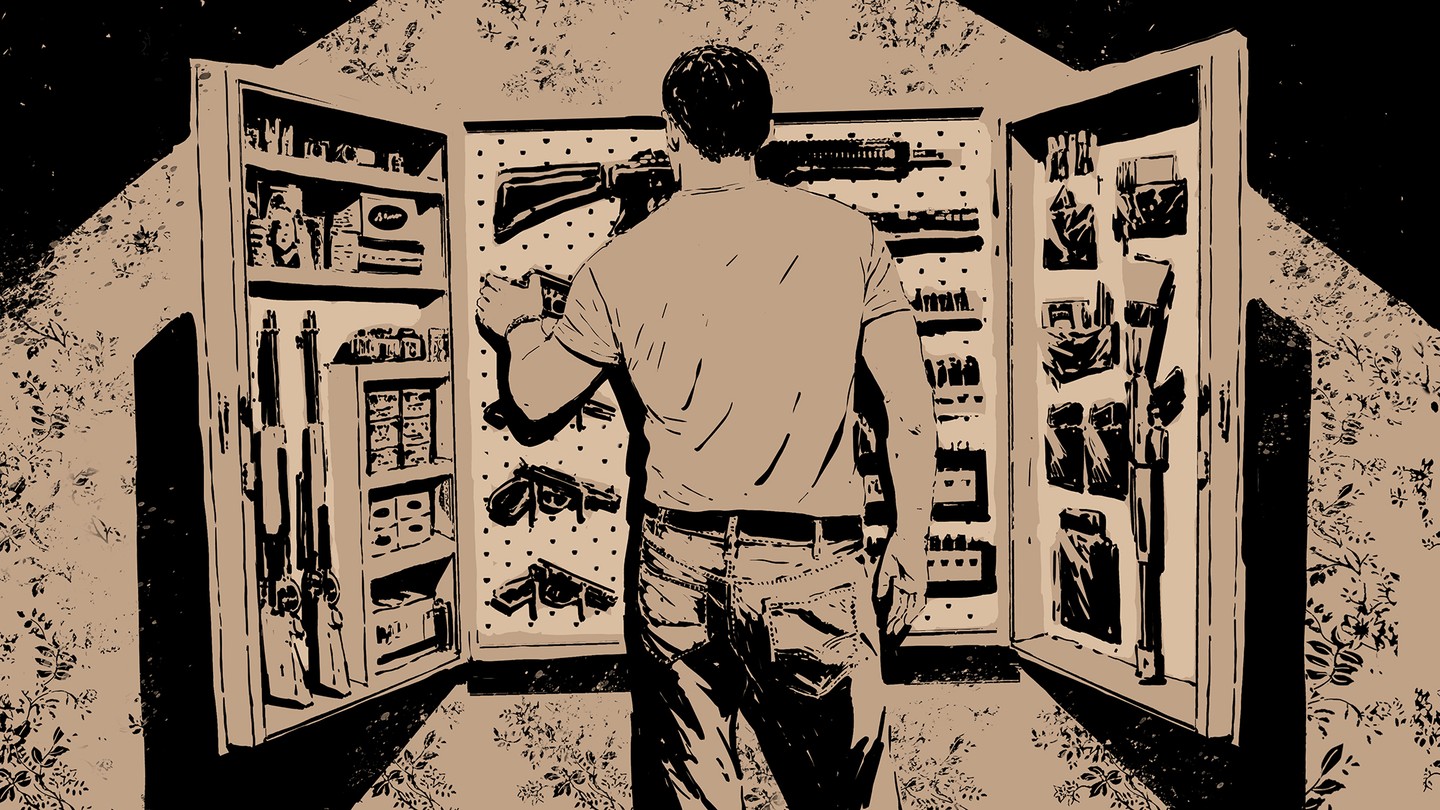The image is a detailed, sepia-toned illustration reminiscent of comic book art, featuring a man standing with his back to the viewer. He is depicted in beige tones with heavy black inking, wearing a t-shirt, jeans, and a belt. The man, who has short black hair and a stocky build, is reaching out with his left hand to touch one of the many pistols inside a large, open wall-mounted cabinet. The cabinet, lined with various firearms including pistols, rifles, shotguns, and boxes of ammunition, contrasts sharply with the floral-patterned wallpaper surrounding it. The wallpaper, predominantly in beige with black splotches and floral designs on the edges, adds an interesting juxtaposition to the weapons of destruction contained within the cabinet. The overall color palette includes shades of black and a pinkish-gray hue, enhancing the monochromatic and illustrative quality of the image.